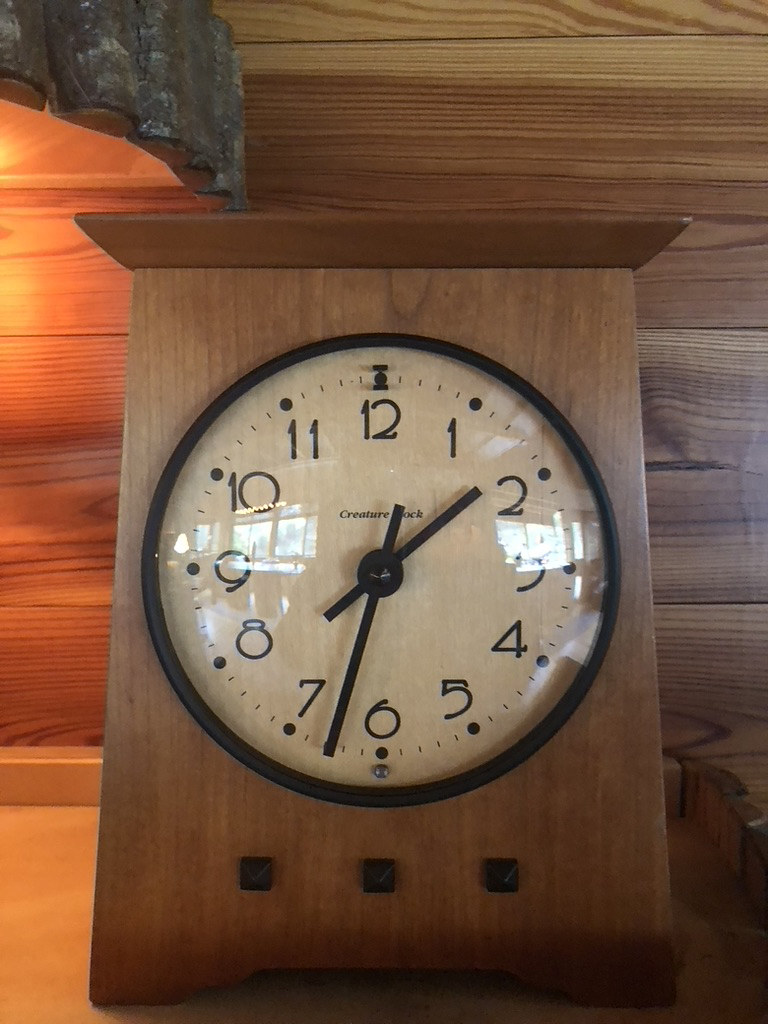A beautifully crafted wooden clock stands elegantly with its rich brown wood body and tall, rectangular shape. The top of the clock tapers gracefully into a pointed trim, giving it a distinct and polished look. At the bottom, a small carved section provides a decorative touch, though it serves little functional purpose and often traps dust. Beneath the clock face, three black square buttons are aligned in a neat row. The clock face itself is bordered in black, with a white center that hosts slender black hour and minute hands. Each hour is marked by black numerals from 1 to 12, accompanied by a black dot above each number, and four small dashes between each numeral for precise timekeeping. The back wall behind the clock is also made of brown wood, adding to the rustic charm of the overall setting. A warm, glowing light from a lamp made out of cut logs illuminates the top left corner, casting a cozy ambiance over the scene.